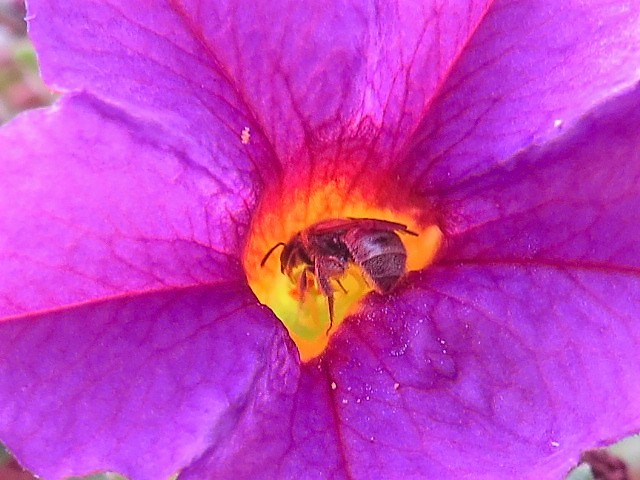In this close-up rectangular photograph, we see a vivid shot of a singular flower and a bee. The flower, which may be a petunia, dominates the image with its striking bright purple petals adorned with hot pink veins. The center of the flower features a bright yellow stamen, almost resembling a fiery orange hue. A bee is situated at the core of the blossom, fully immersed and appearing to gather nectar or pollen. The bee doesn't exhibit the typical yellow and black stripes; instead, it seems to be more of a solid brown color, possibly due to the lighting. The background is subtle, with hints of green in the upper left corner, likely from distant grass or leaves. The primary focus, however, remains on the interaction between the bee and the vibrant flower.